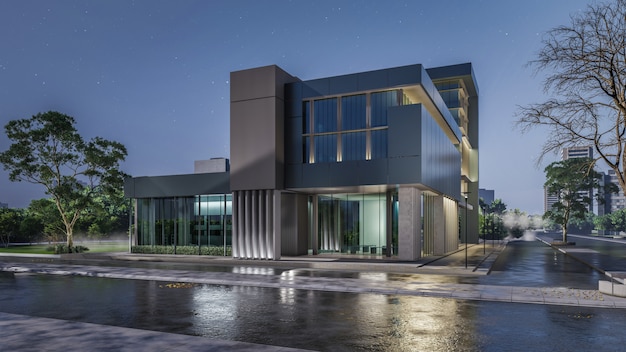The image depicts a modern, city scene with a newly built, three-story building as the central focus. The structure is contemporary, featuring gray and silver tones with expansive floor-to-ceiling glass windows. The building has a clean, minimalist design, possibly suggesting it could be a bank or another professional establishment, though no signs indicate its purpose. In the foreground, the sidewalk appears wet as if it had just rained, contributing to the fresh appearance of the city block.

The background reveals a clear blue sky, which becomes whiter towards the right side of the image. Surrounding the building, there are other architectural elements and natural features. A large tree with green foliage stands to the left of the building, accompanied by other green trees behind it. On the right side, a bare tree with brown or gray branches adds contrast. Additional buildings are visible in the distance, behind another tree with green leaves and similarly colored branches. The white structures add to the urban atmosphere.

The bottom left corner shows a sidewalk, transitioning into what appears to be a gray driving area or street, which separates into another sidewalk covered with whitish rocks. In front of the building, there are small bushes, and indoor houseplants in green pots can be seen through the windows, adding a touch of greenery to the scene. The house itself, though modern, complements the overall setting with its detailed design and surrounding natural elements.